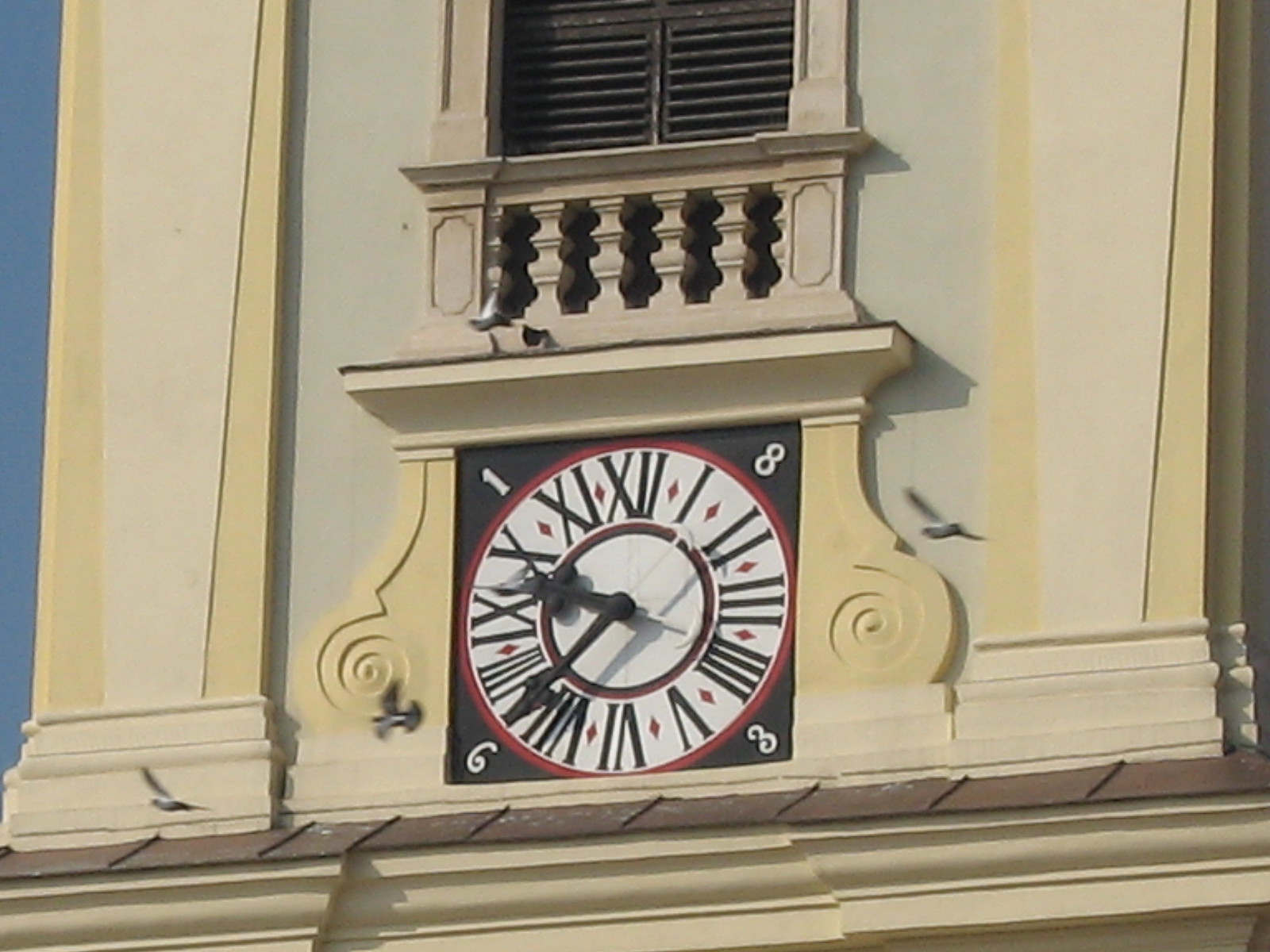This is a medium-quality, landscape-style photograph zoomed in on an old, slightly faded yellow-cream building with a prominent clock. The building appears run-down, with its color fading over time. The clock, encased in a black square outline with a white face, features large black Roman numerals and hands. Surrounding the clock is intricate stonework, including flourished concrete framing, a faux balcony, and fake shutters. In the background, there are also some blurred pigeons flying across. The time on the clock seems to be approximately 7:50. Additionally, the corners of the clock face include angled white numbers 1, 8, 3, and 6, which might signify the year 1863.